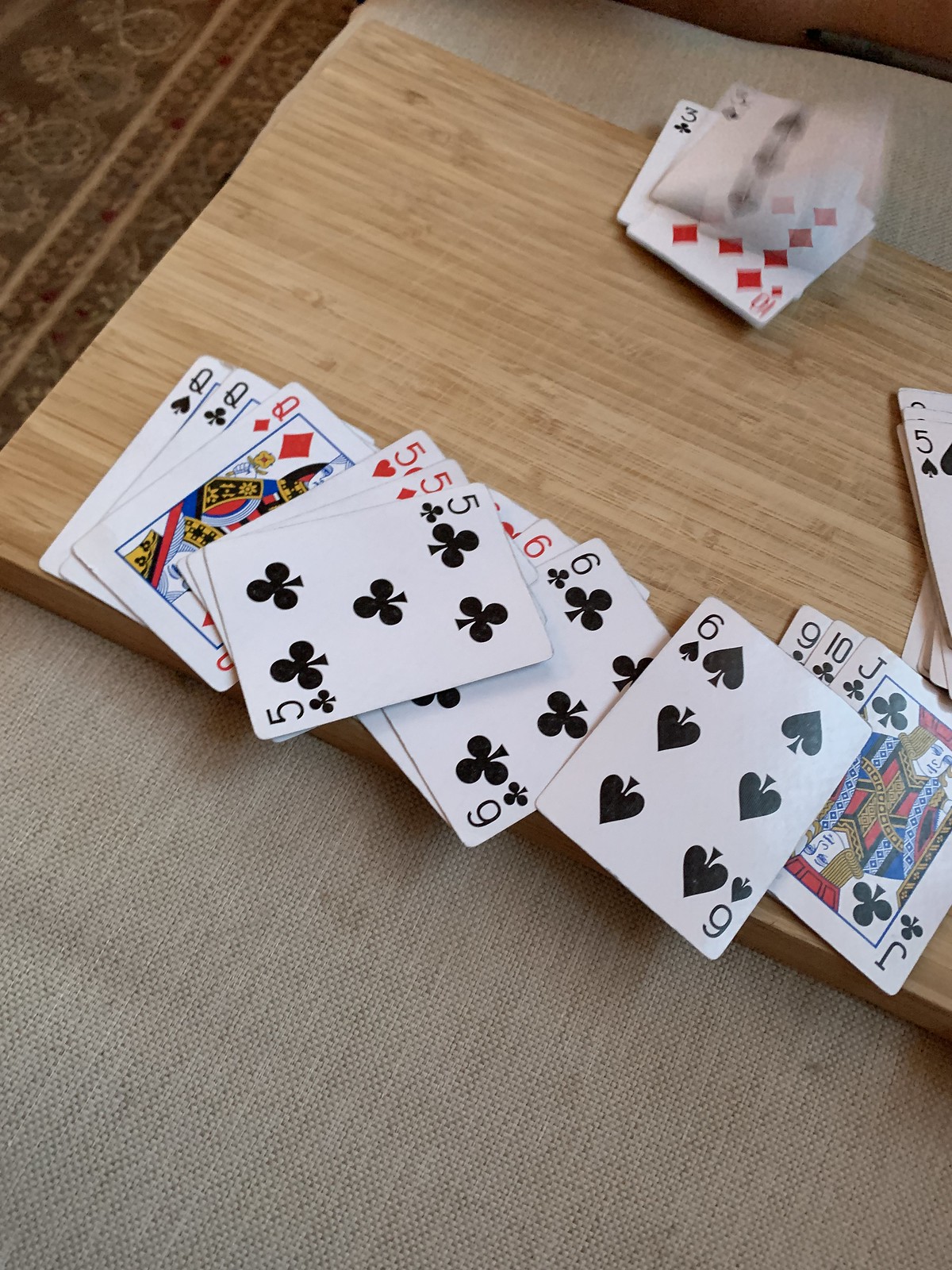This indoor photograph captures a dynamic array of standard playing cards arranged on a light wooden surface, possibly part of a small desk or plank set atop a light beige-gray linen fabric, presumably a sofa. The cards are scattered in a row, angled diagonally downward to the right. A neat stack of cards lies at the bottom right, topped with a Jack of Clubs. Above this, another small deck exists near the top right corner, with an Ace of Spades appearing blurry in mid-air as if someone is in the act of throwing it onto the pile. The light wooden surface contrasts with an oriental rug, visible in the upper left corner, featuring a red, black, and beige pattern. All the cards have white backs, lending a clean, cohesive look to the arrangement.